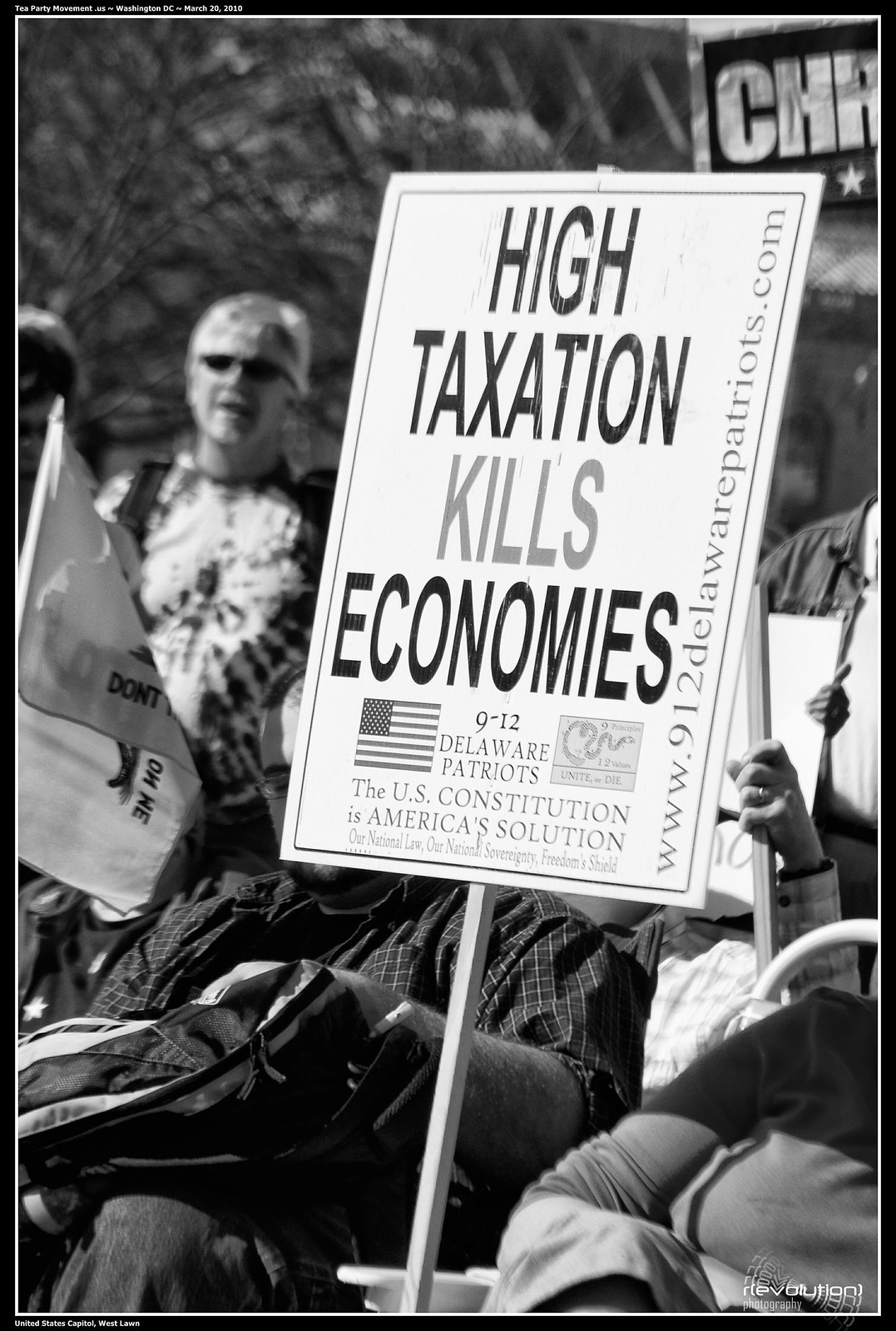The image appears to be a vintage black-and-white photograph taken during an election-related event or protest. It has a black border with a thin white inner border. There are small, unreadable white words at the top of the black border. The scene captures a group of people sitting and standing, many of whom are holding signs. The central focus is a large, square, white sign with bold black capital letters that reads, "HIGH TAXATION KILLS ECONOMIES." The word "KILLS" is notably in light gray. Accompanying the text are an American flag and a "Don't Tread On Me" flag. The sign also includes the message, "9-12 Delaware Patriots. The U.S. Constitution is America's Solution," and vertically along its side, it states, "www.912delawarepatriots.com." At the bottom edge, additional text reads, "Our national law, our national sovereignty, freedom shield." Another small fabric "Don't Tread On Me" flag is seen blowing in the wind, further emphasizing the protest's patriotic themes.